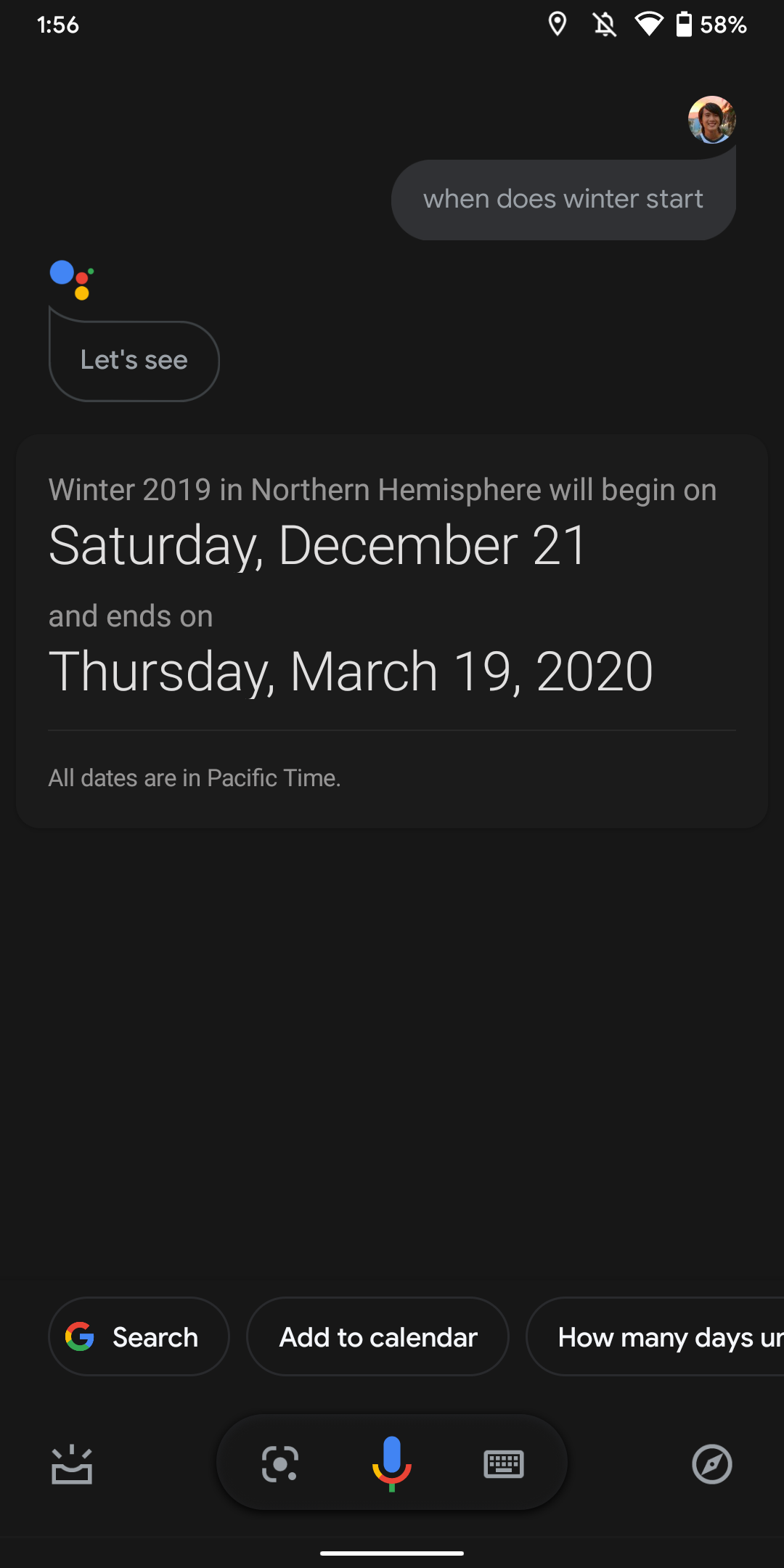A screenshot captured at 1:56 p.m. displays a smartphone interface with 58% battery remaining. The device is operating in dark mode, which reduces eye strain by using a black background. The focal point of the screenshot is an interaction with an AI chatbot, presumably Google Assistant. The user has queried about the start of winter, to which the chatbot responds: “Winter starts on Saturday, December 21st and ends on March 19th.” The concise exchange highlights the utility of AI in providing quick, informative responses to seasonal questions.